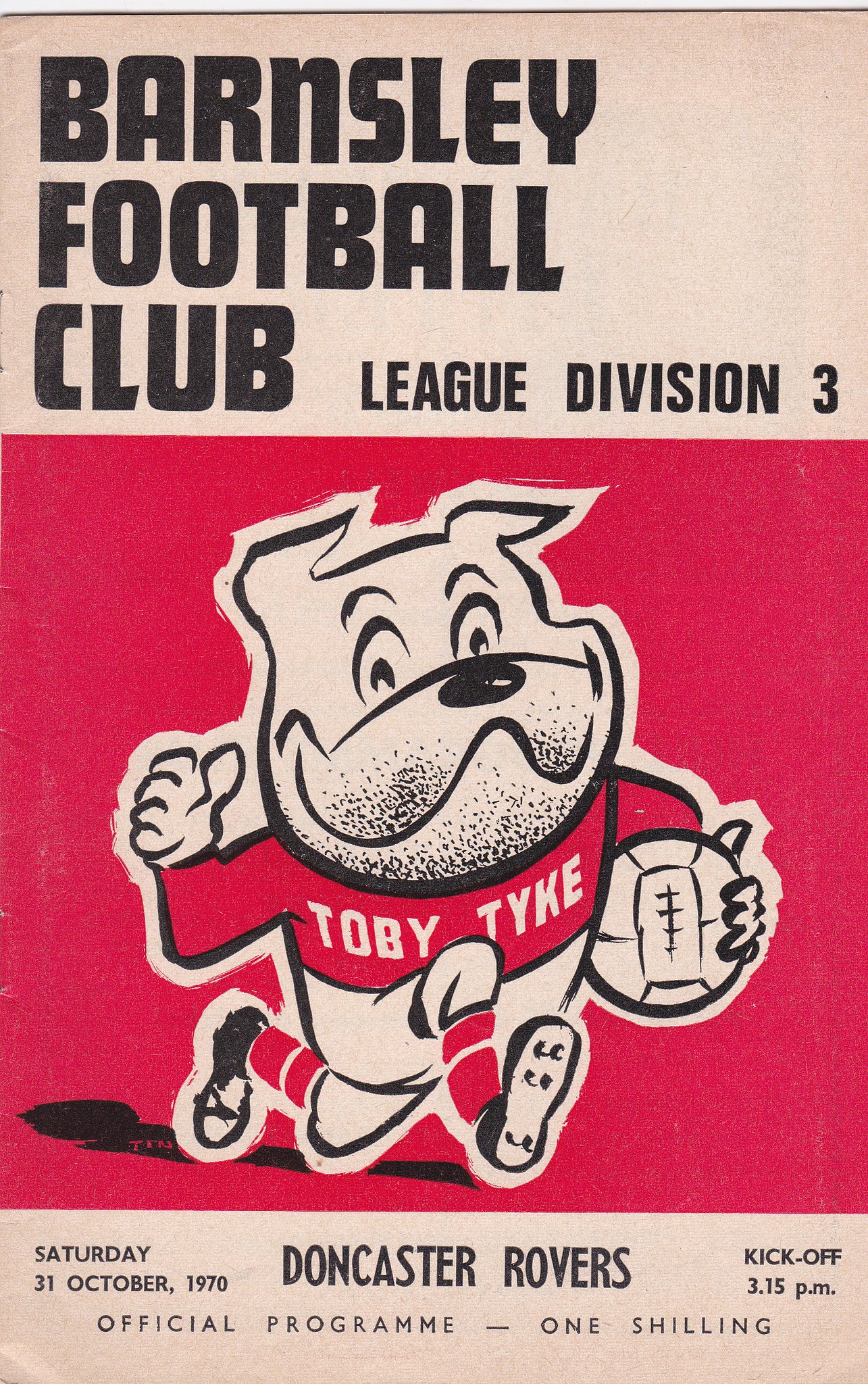This vertically oriented, rectangular advertisement for the Barnsley Football Club features a nostalgic design from 1970. At the top, set against a light flesh-colored background, bold black text announces "BARNSLEY FOOTBALL CLUB," with slightly smaller text to the right reading "LEAGUE DIVISION III." Below this header, a square red section showcases a cartoon mascot—an energetic bulldog named Toby Tyke, depicted in a vintage, stylized manner. The bulldog runs to the right, holding a white soccer ball in one hand. He sports a red shirt emblazoned with "Toby Tyke," long red sleeves, white shorts, red socks, and black shoes. His ears point backward and his left arm is raised high, casting a shadow behind him. The bottom of the poster features vital event details in black text: "Saturday 31 October 1970," "Doncaster Rovers," "kick-off 3.15 p.m.," and "official program one shilling." The overall design exudes an old-school, cartoonish charm, reminiscent of a bygone era.